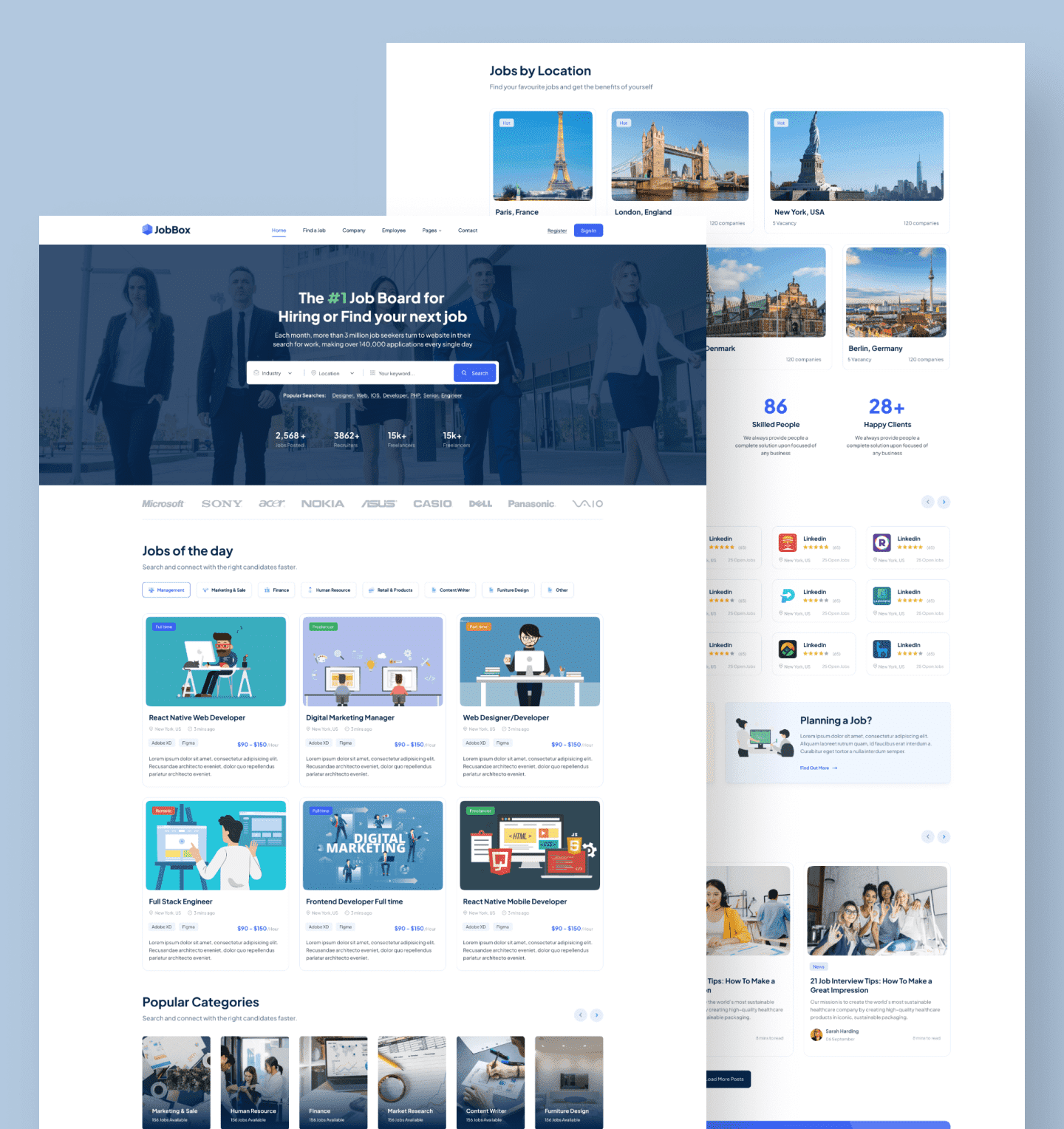The image depicts a job search website interface in detail. The background features the section "Jobs by Location," which lists various cities and associated job information, though this section is partially obscured by an overlay. 

The overlay prominently declares, "The Number One Job Board for Hiring," followed by the prompt "Find Your New Job." Beneath this is a search bar for users to input their job search criteria. 

Additionally, the "Job of the Day" section is highlighted, showing a caricature of a person working at a white desk. This character has dark hair and is dressed in black pants. 

Subsequent sections also feature caricatures: One showcases two people working at their computers, one in gray attire and the other in red. Another caricature depicts a person standing at a white table with a computer, holding a coffee cup, dressed entirely in black.

Further down, there's an illustration of a woman with short black hair wearing a white shirt, standing and looking at a screen in front of her. 

The bottom part of the interface presents a blue screen with five images of a man dancing, dressed in all blue, and mentions "Popular Categories."